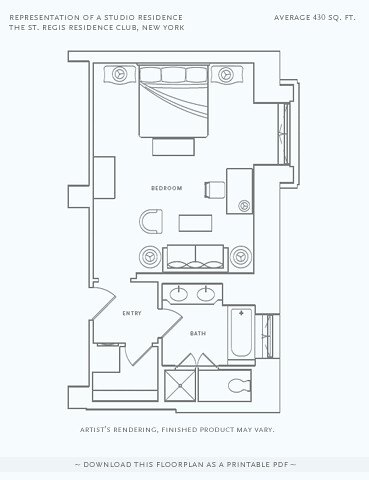This image is a representation of a studio residence at the St. Regis Residence Club in New York. The overall image quality is somewhat blurry and not optimal, but it provides a general layout of the floor plan. The floor plan can be downloaded as a printable PDF, as indicated by a text prompt. The top left corner of the image reads "Representation of a Studio Residence, the St. Regis Residence Club, New York", while the right side notes an average size of 430 square feet. The bottom of the image features the disclaimer: "Artist's rendering, finished product may vary."

The floor plan depicts a vertically arranged studio apartment, comprising a single-room living and sleeping area, along with a bathroom. The sleeping area shows a bed adorned with three pillows and a small footstool at its base. Flanking the bed are two end tables, each topped with a lamp. Adjacent to the bed, there is a small desk with a chair, and nearby, a sofa and an additional chair suitable for TV viewing, accompanied by two small round tables with lamps.

The bathroom features a bathtub and two sinks, with a window providing natural light. Additionally, the bathroom includes a separate enclosed area for the toilet, accessible through its own door. The layout maximizes functionality within the 430-square-foot space, offering comfortable living amenities.